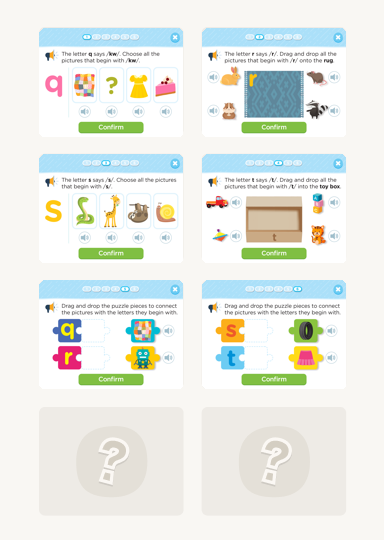A carefully arranged set of images, depicted in multiple orderly squares, each accompanied by a "confirm" button. Starting from the top:

1. **First Square:**
   - Contains a 'P', a quill, a question mark, a yellow dress, and a pink slice of cake, each with a circular volume icon beneath them.
   - Underneath these items, the word "confirm" is prominently displayed.

2. **Second Square (to the right of the first):**
   - Displays a rabbit, a mouse, another rabbit, and possibly a cat, also with a confirm button beneath.

3. **Third Square (below the first two):**
   - Features an 'S', a snake, a horse, and a snail, all accompanied by volume circles, with the word “confirm” situated below.

4. **Fourth Square:**
   - Shows a truck, a spinning top, some blocks, and a cat, highlighted by a prominent 'T' in the center of the square.
   - A brown box is also part of this set, followed by the word "confirm".

5. **Fifth Square (below the fourth):**
   - Includes an 'S', a 'T', a tire, and a pink skirt, all depicted as pieces of a puzzle, with the word "confirm" beneath.

6. **Sixth Square (to the left of the fifth):**
   - Contains a 'Q', an 'R', a variety of small squares, and a robot, also as puzzle pieces, with "confirm" written below them.

7. **Two Gray Squares (below the sixth):**
   - Each featuring a question mark, shaded in gray, without any additional text or imagery.